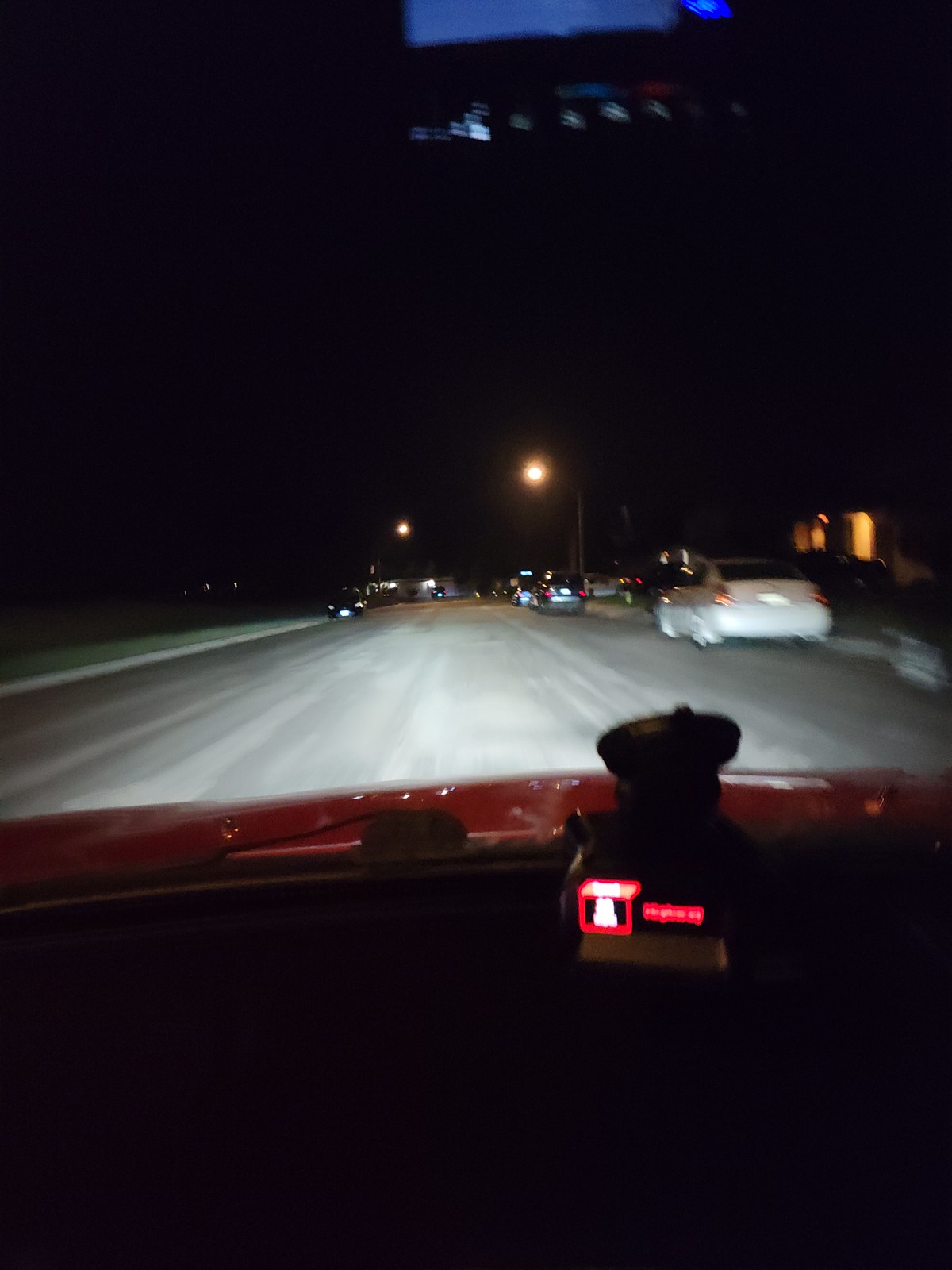The photograph, taken at night, offers a view from inside a vehicle. Mounted on the dashboard is a device with a screen displaying red figures. The vehicle's hood is partially visible, revealing a red car driving down a street illuminated by traffic lights—two of which are visible. In the distance, a lit-up structure, possibly a house, can be seen. Directly ahead of the vehicle, a white car leads the way, followed by several more vehicles farther up the road. The night sky is pitch black, and the car is about to pass under a structure that appears to be a road or interstate sign. The top portion of the sign is a royal blue color, and it is surrounded by other lights, suggesting it may be a billboard advertising something. The scene captures the essence of nighttime driving on a bustling street.